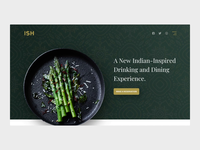This image is a screenshot that appears to be from a mobile browser, cropped to show only a portion of an advertisement or website. The overall background is gray, framing a smaller, central section. This central section features a very dark green rectangle that seems to be the hero section of a webpage.

At the top left of this dark green rectangle is a golden logo, which is too small to identify clearly. Opposite the logo on the top right, there is a navigation menu, but the text is unreadable due to the small size. Below this, occupying the main part of the hero section, is an image of a dark cast iron pan containing asparagus, possibly cooked with oil and herbs.

To the right of the cooking pan, there is a textual heading in white letters that reads, "A new Indian-inspired drinking and dining experience." Beneath this heading is a yellow button with white text, which is illegibly small. The entire dark green rectangle is bordered by a tiny white sliver at the bottom, transitioning into the surrounding gray background.